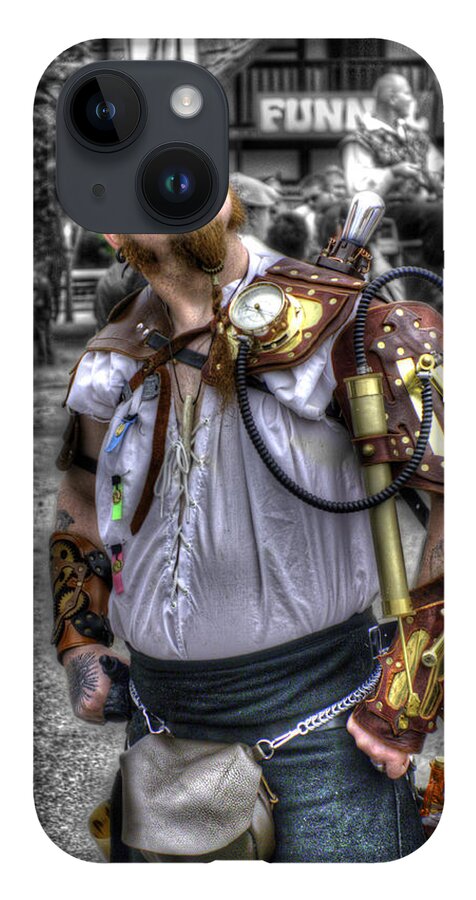This vertically aligned, rectangular image with rounded edges showcases a phone case featuring a detailed depiction of a man adorned with various steampunk-esque gear and gadgets. In the upper left corner of the case, the iPhone's dual camera lenses are positioned to resemble the man's eyes—one lens lit up in a light blue hue and the other in a darker blue, with small, distinctive dots in the opposing corners. The individual sports an orange goatee and wears a white, old-fashioned shirt, reminiscent of 1700s or 1800s sailor attire, fastened with ties rather than buttons. His ensemble includes dark pants and a chain belt with an attached pouch, resembling a fanny pack. His arms, covered in black and gold armor reminiscent of historical battle gear, extend with visible hands—one bearing a tattoo. The right shoulder of the armor features a steam gauge-like dial, adding to the steampunk aesthetic, while the left wrist is adorned with a simple guard. Numerous small, bug-like details with straps adorn the left side of his shirt. The man's face is partially obscured by the camera lenses, adding an element of intrigue, while the word "FUNN" is faintly visible in the background, enhancing the whimsical, cosplay vibe of the image.